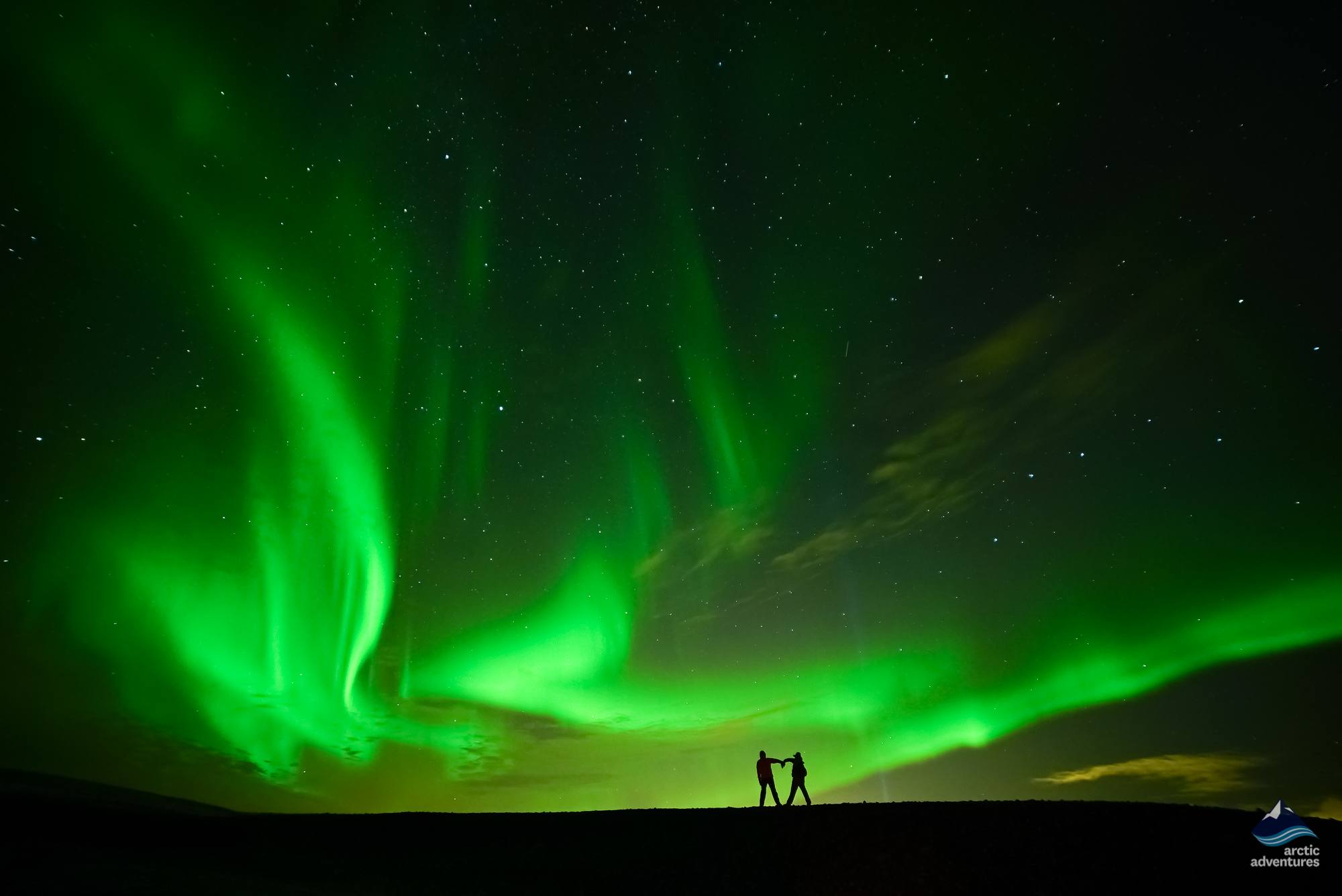In the image, a vivid, neon green sky stretches across the night, illuminated by the striking patterns of what appears to be a green aurora with hints of yellow-green shadings. The contemporary, artsy style is set against a dark, almost black sky, interspersed with a few bright stars. Silhouetted prominently in the foreground are two people whose figures are connected in an elongated heart shape formed by their joined hands and slightly separated legs, standing on a relatively flat, dark surface. In the bottom right corner, a small watermark with a mountain and blue wave logo reads "Arctic Adventures," suggesting a link to Arctic exploration. This captivating image beautifully contrasts the eerie, vibrant glow of the aurora with the stark silhouettes, making it a potential poster-worthy representation of a Northern Lights adventure.